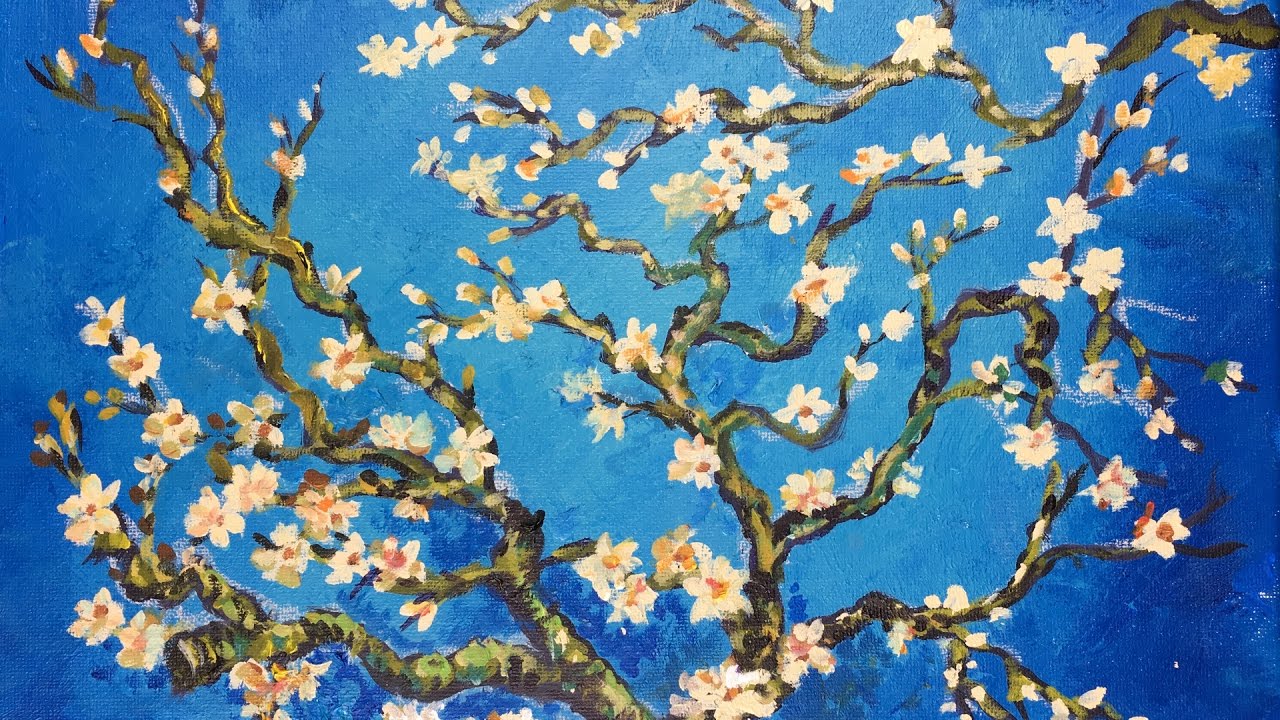The painting depicts a tree adorned with delicate white blossoms, each featuring five to six petals and a yellow to orange center, resembling daisies. The tree's branches, which are a mix of green and brown hues, start from a central stalk and branch out in a Y shape, splitting further into smaller, thinner branches that spread across the canvas. On the right top side, there is another branch, possibly from a different tree, that also carries these blooms. The background of the painting transitions from a deep blue around the edges to a lighter blue at the center, suggesting a sky. The branches are uneven, curved, and scattered throughout, creating a dynamic composition. The overall style evokes traditional Japanese paintings, emphasizing the natural beauty of the scene. The tree is depicted in a side view, highlighting its intricate branching structure and numerous blossoms, making it a visually captivating artwork.